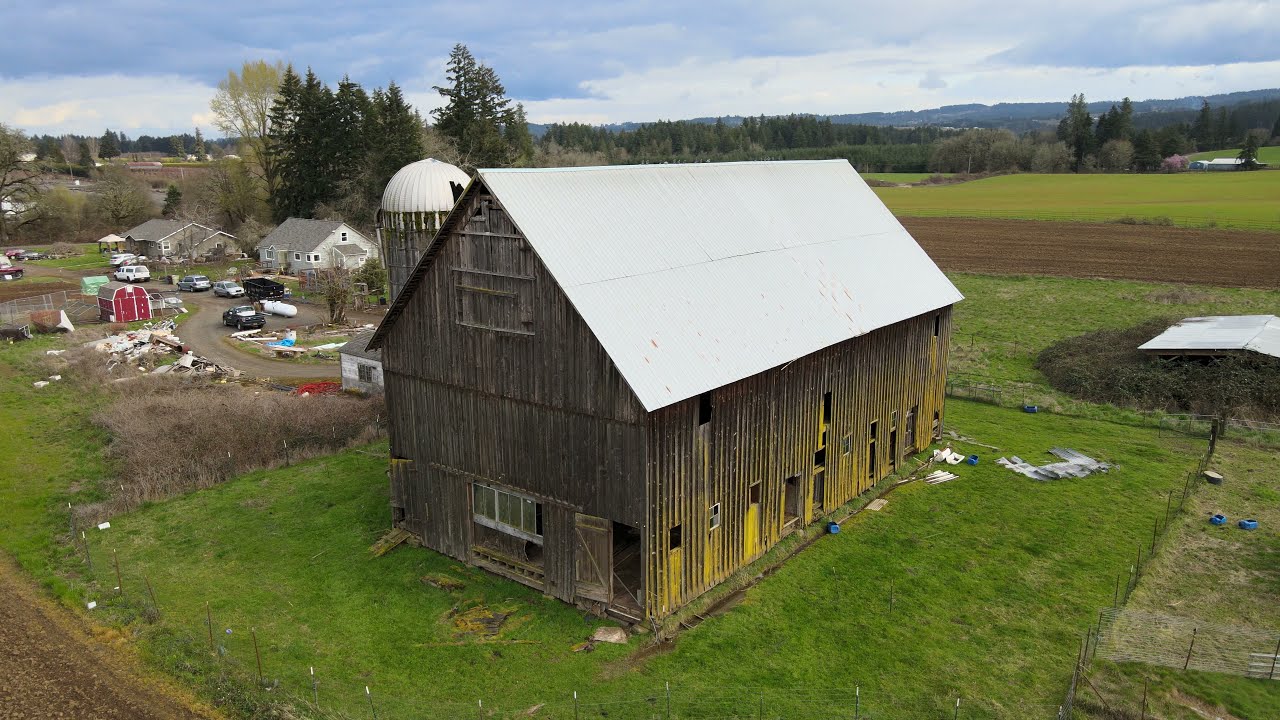The image is a horizontally aligned rectangular picture taken from slightly above ground, offering a detailed aerial view of an old, worn barn at its center. The barn, characterized by its dark, weathered wood, features a faded yellow tint near the bottom edges. Its roof is a solid, silvery white, sloping down to meet the aged wooden sides. Adjacent to the barn on the left is an old silo with a silver top, blending seamlessly with the barn's dilapidated appearance.

The barn stands amidst a patch of short, green grass, interspersed with scattered debris, blue and white objects, and patches of browning weeds. In the background, a horizon of green trees under a partly cloudy sky sets the scene. The sky itself is painted with gray and white clouds, adding a somber tone to the picture. To the left, a small community appears, featuring a few houses, some vehicles, a small red outbuilding, and a dirt path winding through. Further in the background, rows of farm fields and tilled dirt stretch out, depicting a rural landscape dotted with trees and additional farm structures.